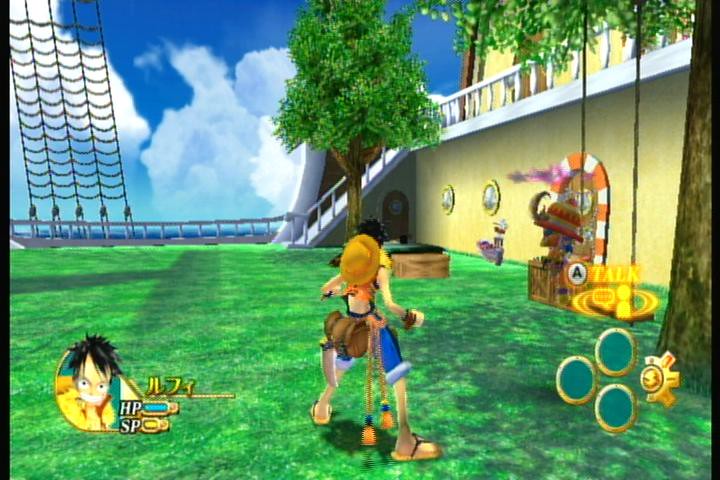The image appears to be a detailed screenshot from a video game. Positioned in the center bottom half of the frame, the main character stands in a wide, laid-back stance on a green grassy field. He is dressed in blue jean shorts, a long fluffy white collar ending just above his knees, flip-flops, and a hat that is strung behind him rather than on his head. Fronted by a tree with a brown trunk and green leaves, the setting is completed by a blue sky filled with white clouds in the distant background. 

The scene seems to take place on a large ship, implied by the presence of ropes, a rope ladder on the left-hand side, and round porthole-like windows visible in the background. A distinctive arched doorway with orange and white stripes is also part of the setting.

On the bottom left-hand corner of the image, there is a circular player icon featuring the character’s face with black hair, white eyes, and what looks like a yellow outfit inside an oval portrait. Next to this icon are power indicators, with the character's HP (highlighted by a blue bar) and SP (highlighted by a yellow bar), topped with some Asian characters. In the bottom right corner, there are three circular spots with a golden outline and green interior, along with another icon that has a three-pronged gold pattern enclosing a small golden coin.